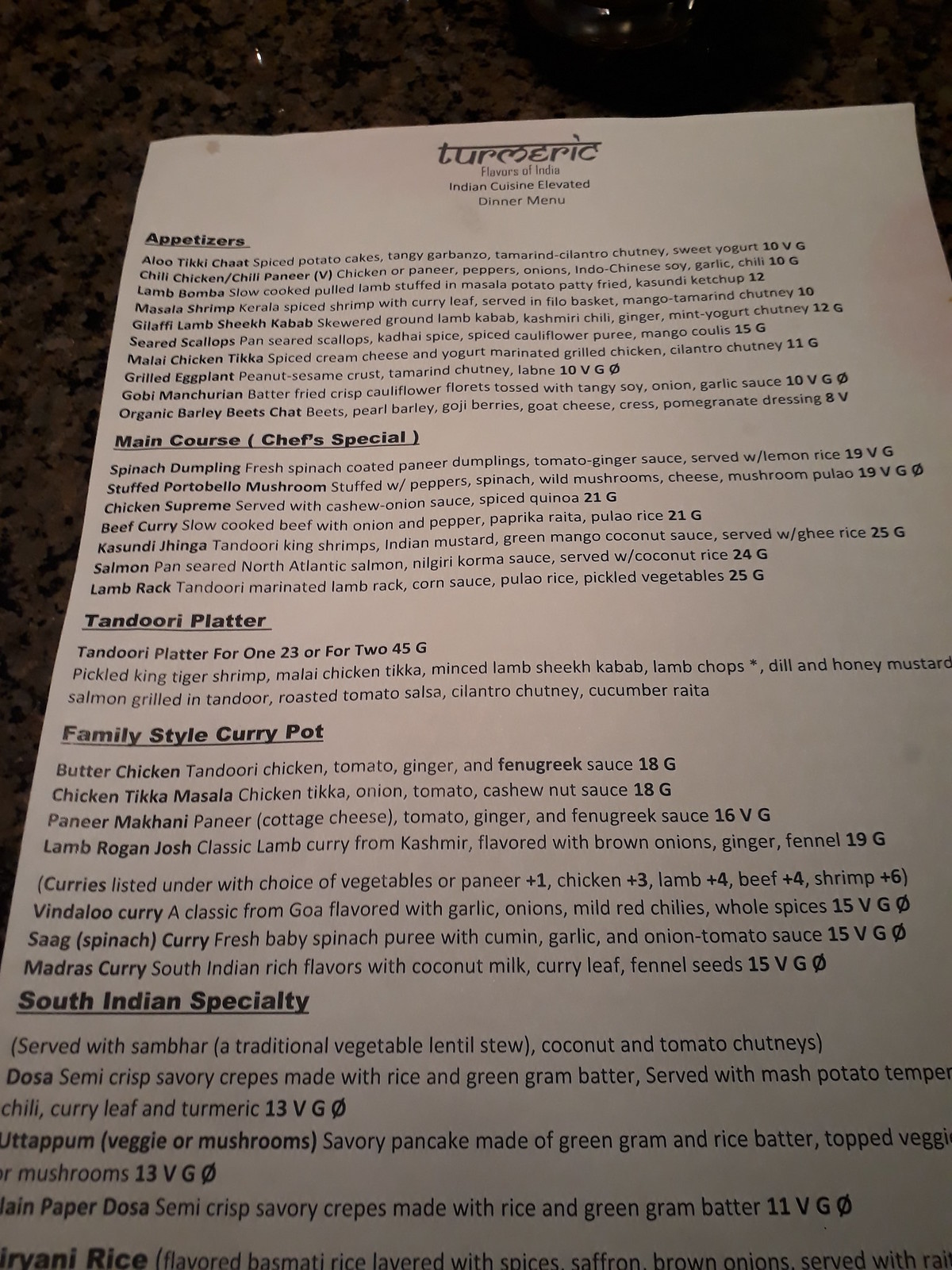This vibrant color image showcases the elevated dinner menu of "Turmeric Flavors of India," an Indian cuisine restaurant. The menu is divided into distinct sections, starting with appetizers that include a diverse selection such as Aloo Tikki Chaat, Chili Chicken or Chili Paneer, Lamb Bamba, Masala Shrimp, Gilafi Lamb Seekh Kabob, Seared Scallops, Malai Chicken Tikka, Grilled Eggplant, Gobi Manchurian, and Organic Barley Beets Chaat.

Moving on to the main courses or chef specials, the options are equally tantalizing: Spinach Dumplings, Stuffed Portobello Mushroom, Chicken Supreme, Beef Curry, Kasundi Jhinga (a flavorful shrimp dish), Salmon, Lamb Rack, and a Tandoori Platter available for one or two persons.

Lastly, the menu features a family-style Curry Pot section, including delectable choices like Butter Chicken, Chicken Tikka Masala, Paneer Makhani, and Lamb Rogan Josh. Additional curry dishes available are Bindaloo Curry, Saag Spinach Curry, and Madras Curry.

The image encapsulates the rich and varied offerings of the restaurant, promising a memorable dining experience with its array of flavors and dishes.